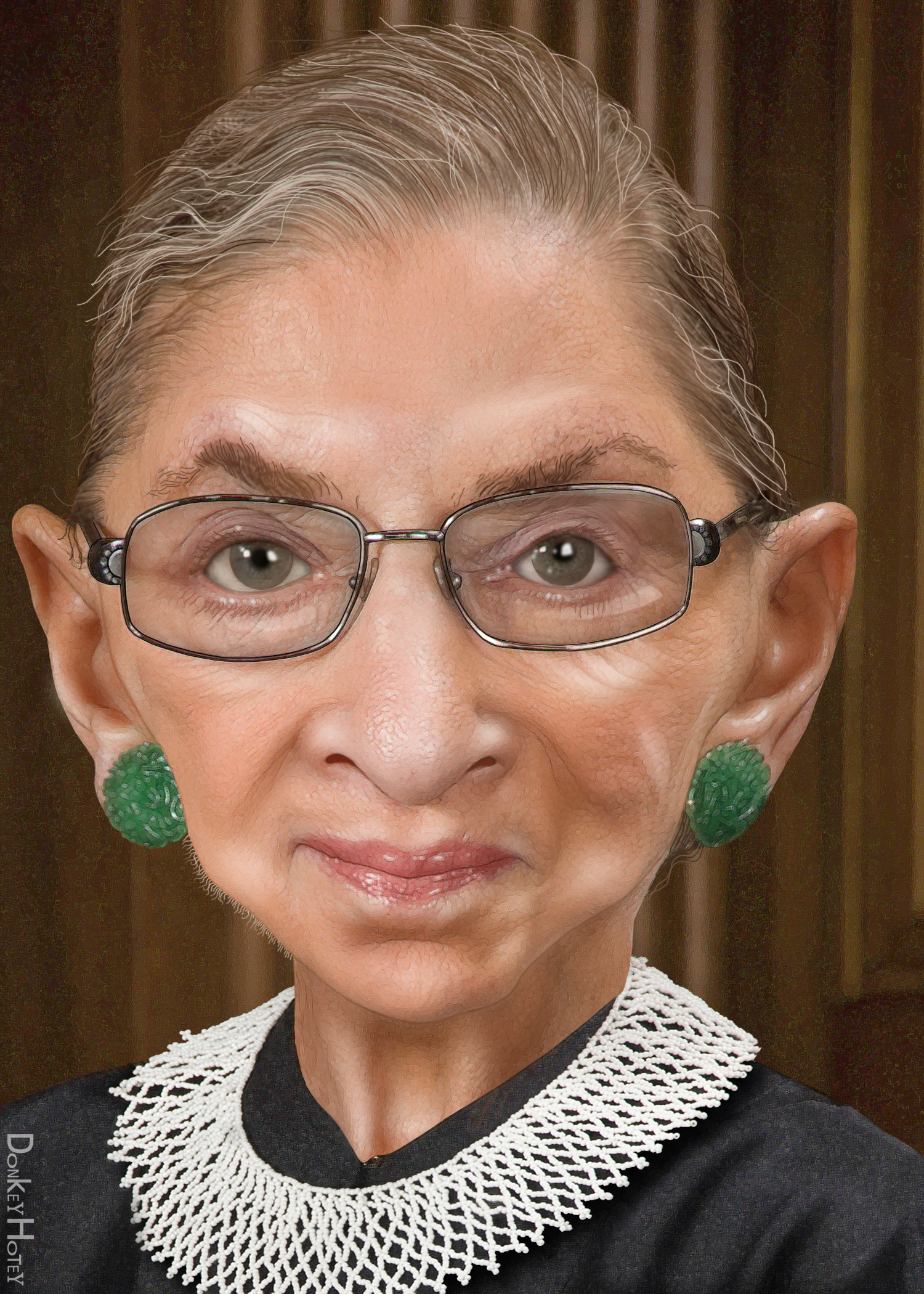The image is a caricature of Ruth Bader Ginsburg, featuring an exaggerated portrayal with an enormously large head. Her distinctive features, such as her eyes, ears, and nose, are prominently accentuated. Ruth Bader Ginsburg is depicted in her traditional judicial garb—a black robe with a very ornate, crochet-like white collar. She has round, large green earrings and wears her stereotypical silver-rimmed glasses. Her hair, which is brown with streaks of gray, is styled up and parted to the side. She has a serious expression on her face. The background of the image appears to be made of a brown wooden panel. In the bottom left-hand corner, there is some barely readable text in white that appears to say "DONKEY HOTEY". The color palette of the caricature includes peach, brown, gray, black, white, green, pink, and various shades of brown.